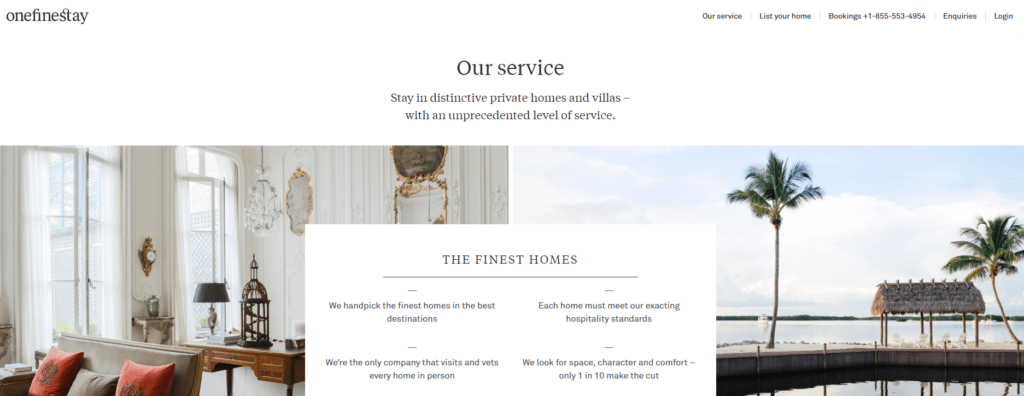The webpage from One Fine Stay, a premium rental service akin to Airbnb, features a sleek and inviting layout. The logo, "One Fine Stay," is prominently displayed in the top-left corner, establishing brand identity. To the right of the logo, a horizontal navigation panel includes several tabs: "Our Service," "List Your Home," "Bookings" (featuring the contact number +1-855-553-4954), "Inquiries," and "Login."

Centrally positioned below the navigation bar, the headline "Our Service" is accented by the description, "Stay in distinctive private homes and villas with an unprecedented level of service." This tagline sets the stage for the rest of the page content, underscoring the exclusive nature of the offerings.

Directly below this, the page visually captivates visitors with two contrasting images. On the left, an interior photograph showcases the elegance and comfort of a well-appointed room within a home or apartment. On the right, a picturesque beach scene, complete with palm trees and a quaint hut, entices those dreaming of a tropical getaway.

Bridging these images, a prominent white square encapsulates the core of One Fine Stay’s philosophy. The text within reads, "The Finest Homes," and further elaborates, "We handpick the finest homes in the best destinations. Each home must meet our exacting hospitality standards. We’re the only company that visits and vets every home in person. We look for space, character, and comfort. Only one in ten makes it." This detailed message highlights the company’s commitment to quality, emphasizing thorough vetting processes and high standards to ensure a luxurious stay for its guests.